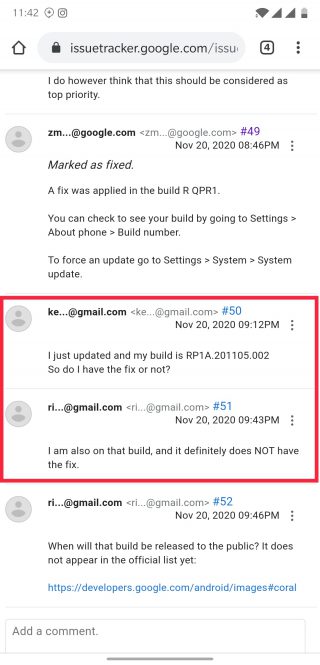The image is a screenshot of a Google Issue Tracker webpage, accessible via the URL issuetracker.google.com. The focus of the screenshot is on a red box highlighting two entries that appear to be user comments or conversations.

Within the box, the first entry is from an email address partially obscured as ke..gmail.com. This comment, marked as number 50, is dated November 20th, 2020, at 9:12 p.m. The user states, "I just updated and my build is RP1A.20.1105.02. So, do I have the fix or not?"

The second entry is a response from a user identified as re, posted approximately 30 minutes later. The response reads, "I also have that build." Both comments are situated in the middle of the image, clearly indicating user discussion concerning a software update build and its associated fixes.